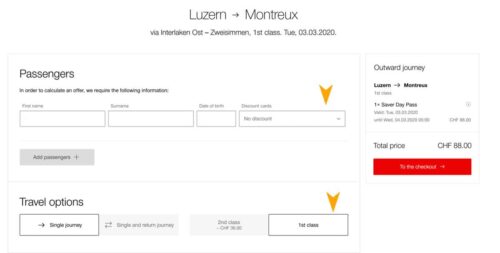The image depicts a web page that seems to be displayed on either a phone or a computer, and it appears to originate from a foreign country. The user on the page is searching for travel information from "Luzern" to "Montreux." The route is indicated with the text “Luzern → Montreux.” The destination names suggest that the locations could be either in France or Canada. The page also mentions the travel date as Tuesday, March 3rd, 2020, which might point to a Canadian origin due to the date formatting. The route details include a leg that mentions travel "via" an unreadable term, noted as "out-z," and specifies first-class travel.

Further down, the webpage has a section for passenger information where users can enter their names, and an option to add more passengers if needed. There is also a section labeled "travel options" for additional preferences or requirements. On the right side of the screen, there is a box labeled "outward journey" that displays the total price of the trip.